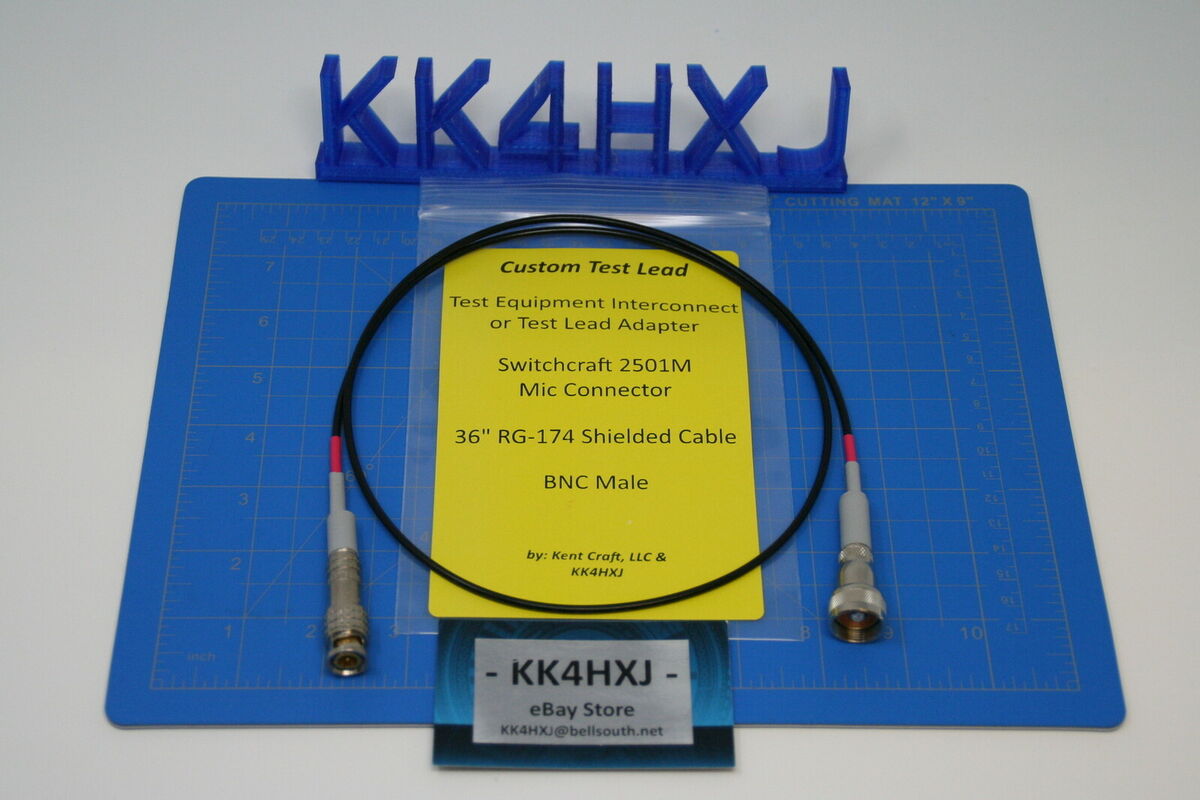The image depicts a product being sold online, set against a white or light gray background. Central to the composition is a blue desk pad with a grid pattern used for measurements. A 3D-printed model number "KK4HXJ" is prominently displayed at the top of the image in blue plastic letters. Below it, there's a business card-like label that reads "KK4HXJ - eBay Store" with the email address "kk4hxj@bellsouth.net."

In the middle of the setup, a small clear ziplock bag contains a custom test lead or test equipment interconnector, described on a yellow label. The label specifies that the item is a "Custom Test Lead, Test Equipment Interconnect, or Test Lead Adapter," with details such as "Switchcraft 2501M Mic Connector" and "36-inch RG-174 Shielded Cable, BNC Male." The coiled test lead cable, approximately three feet long, features a BNC male connector on one end and a female connector on the other, visible through the transparent bag. The entire presentation is neatly organized on the blue grid-patterned desk pad, reinforcing the item's technical and precise nature.